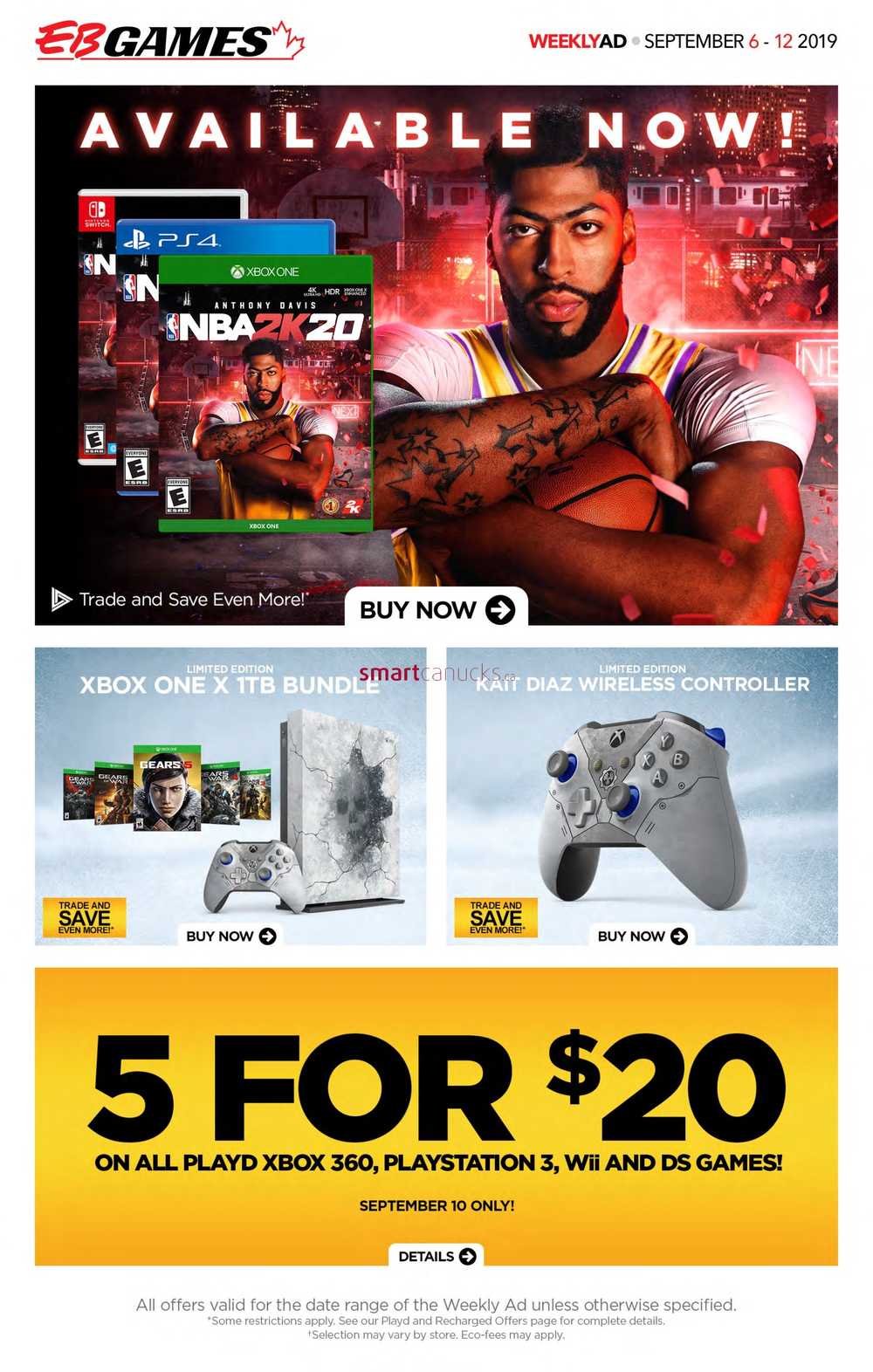This is a detailed caption for the image described:

An intricately detailed weekly advertisement for E.B. Games, spanning the dates from September 6th to September 12th, 2019. Dominating the top half of the ad is a promotional banner for the video game NBA 2K20, featuring prominent imagery of Anthony Davis of the Los Angeles Lakers clutching a basketball, indicating his status as the cover athlete for the game. The ad showcases the game's availability on multiple gaming platforms, including Xbox One, PS4, and Nintendo Switch. Directly beneath this, a bold "Buy Now" call to action is emblazoned in striking black leather against a crisp white background. 

Further down, there is a special promotion for the Xbox One Limited Edition 1 Terabyte Bundle, prominently featuring the Cat Diaz Wireless Controller. The lower section of the advertisement features a gold banner proclaiming a "5 for 20" deal on pre-owned Xbox 360, PlayStation 3, Wii, and DS games, available exclusively on September 10th. Fine print detailing rules and regulations appears at the bottom of the ad, though it is rendered in a small and indistinct font, making it difficult to discern the specifics.